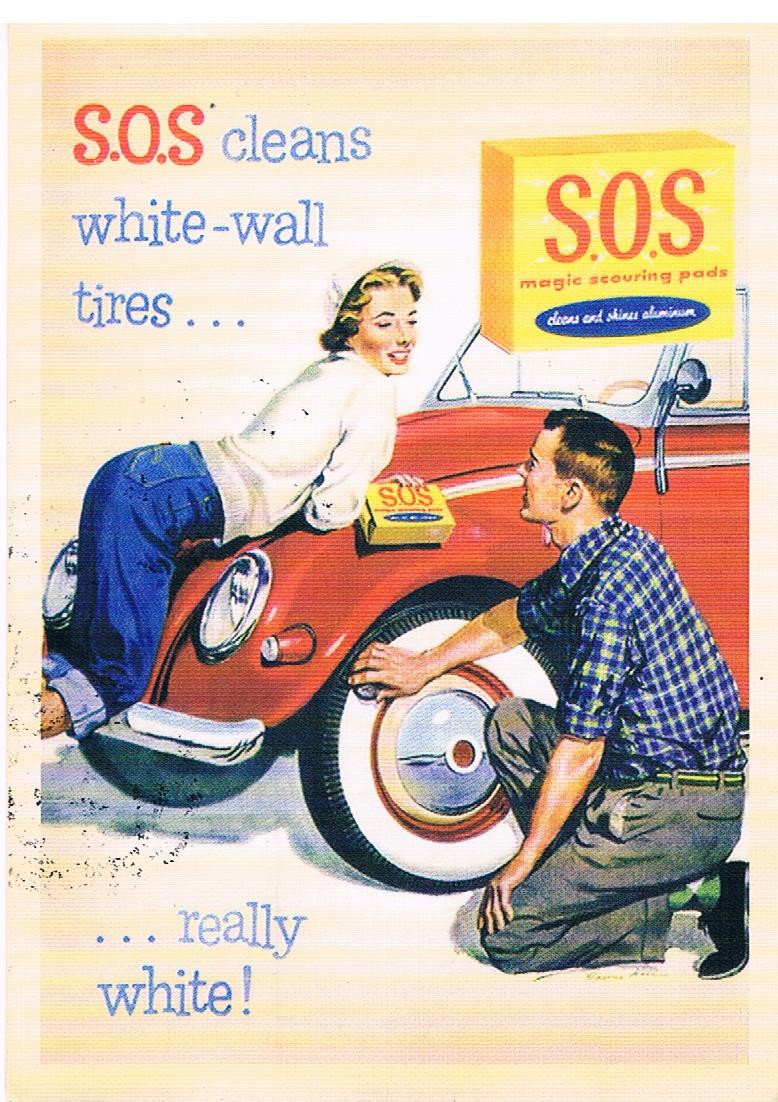This image depicts a vintage painted advertisement with a light beige, almost white background. On the left, bold red letters spell out "SOS," followed by blue text proclaiming "cleans white wall tires..." On the right side, there's an illustration of a yellow box with a red label, containing SOS pads. Below, a vibrant red convertible Beetle is prominently featured. A woman with short blonde hair, wearing a white hat, a white sweater, and rolled-up jeans, is suggestively posed on the car's hood, holding the SOS box. She gazes contentedly at a young man in a blue plaid shirt, gray pants, and black shoes, who is kneeling down and diligently scrubbing the car's tire. At the bottom, in blue text, the ad emphasizes "...really white." The overall scene exudes a nostalgic 1950s ambiance, highlighting the effectiveness of SOS pads in making white wall tires gleam.